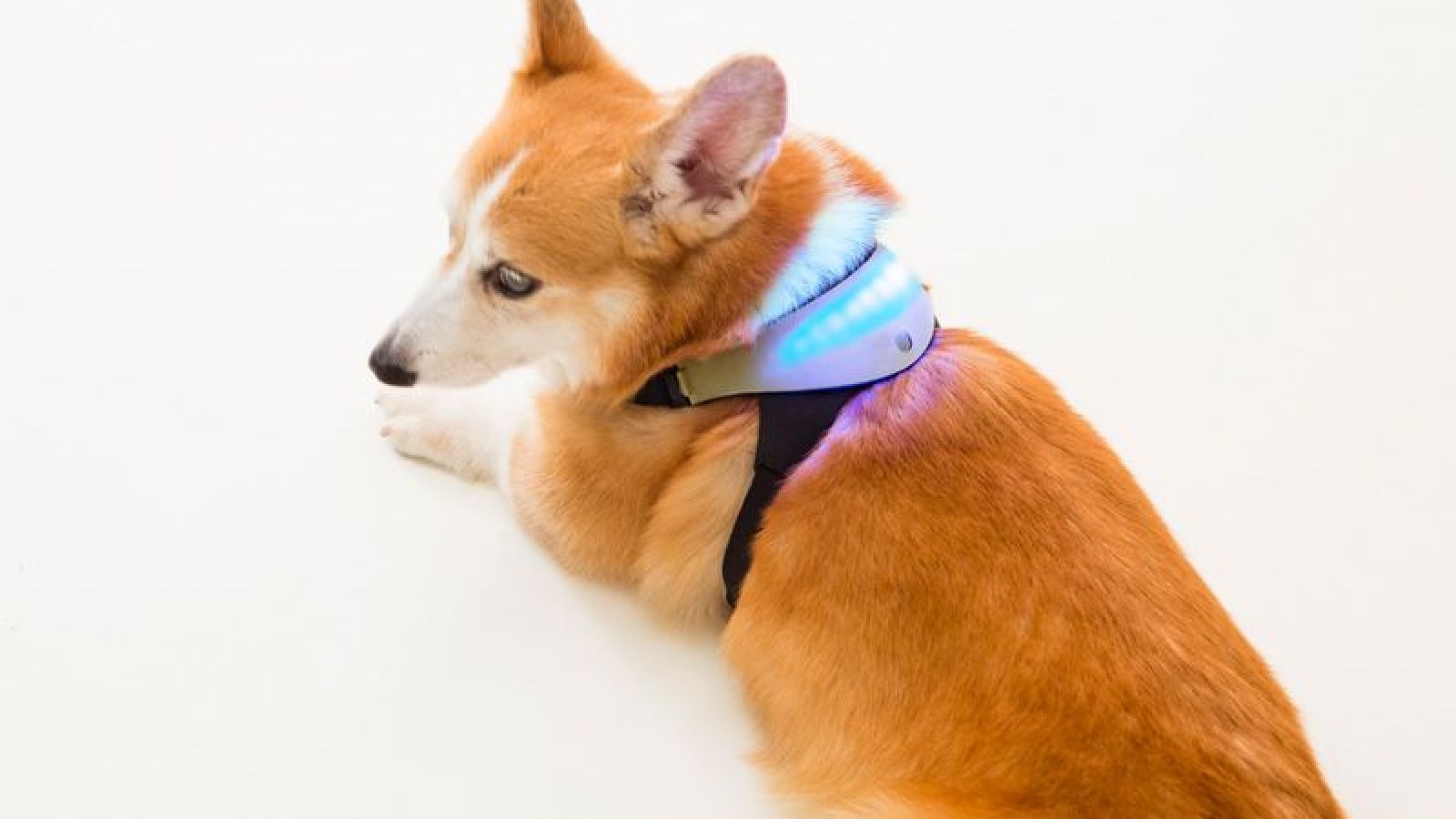A brown dog with light brown fur and white markings on its nose, around its eyes, and on its paws, is laying on a greyish-white, slightly reflective surface. The dog is wearing a smart electronic collar around its neck. The collar, which is white with black straps, has a somewhat spherical device on the back of the dog's neck, featuring blue and white lights that are currently illuminated. The dog is positioned such that its left side is more visible, and it appears to be looking to the left. The background is a clean and clear floor, and there are no other objects in the image.